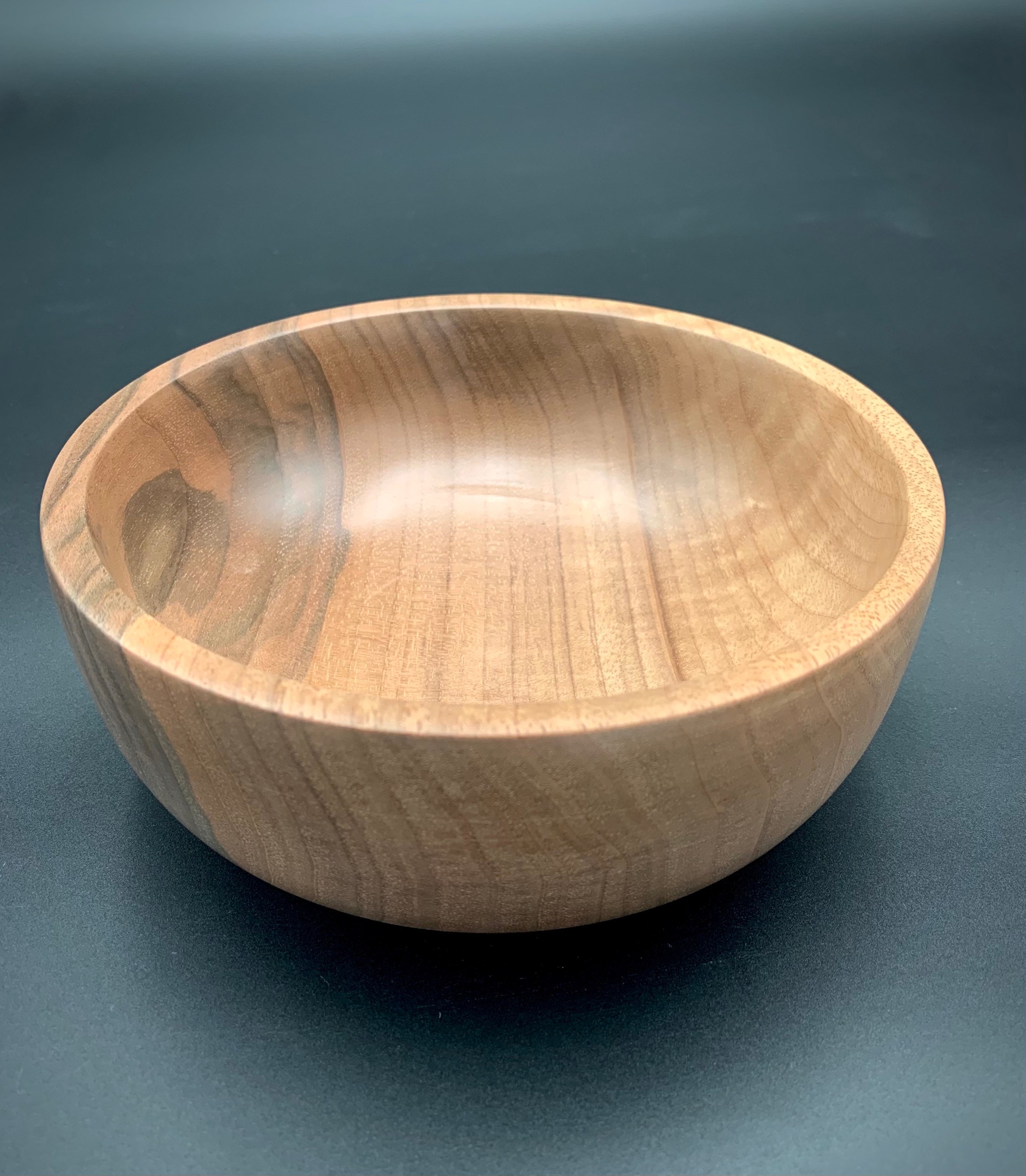Against a dark blue background, a beautifully crafted wooden bowl commands attention at the image's center. The bowl features a light wood interior and rim, with a distinctive dark grain on the left side of its interior, adding a touch of natural variation. The exterior grains are visible, indicating it was expertly carved on a lathe. The bowl is quite substantial, with a thick, flat bottom and sides that rise almost straight up with minimal curvature. It has a subtle sheen suggesting a light oil finish rather than a high-gloss coating. The contrast between the bowl’s light wood tones and the dark blue backdrop highlights the bowl's craftsmanship and the intricate wood grains. The light source from above casts a slight shadow beneath, accentuating its presence as a handmade, smoothly polished piece with hints of light tan and gray, set against a grayish-teal lightbox that intensifies the contrast.